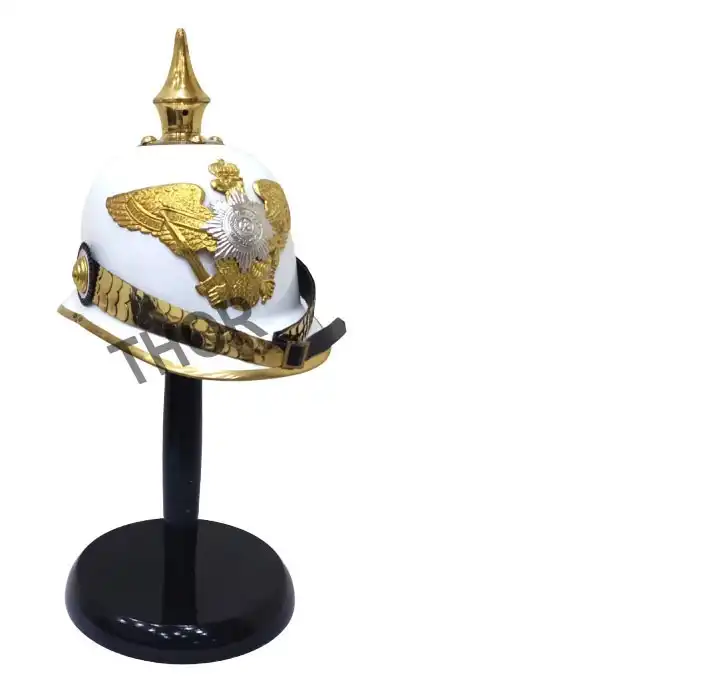Here we have an image of a highly ornate, white military helmet displayed on a sleek black stand against a white background, giving no additional context to its setting. The helmet appears to be an old German or Prussian military helmet, distinguished by its intricate detailing and historical design. At the summit of the helmet is a prominent gold spike, reminiscent of a flagpole's tip. The helmet is adorned with gold accents, including a band encircling the base above the visor and a chin strap. The front of the helmet features an elaborate gold eagle, wings outstretched, clutching what seems to be a spear, with a silver star badge prominently positioned on its chest. Additionally, the eagle bears a crown, enhancing the regal symbolism of this headgear. A gold rim lines the brim, completing the luxurious decoration. The image also includes a watermark reading "Thor" in black letters, suggesting that this piece may be up for sale.